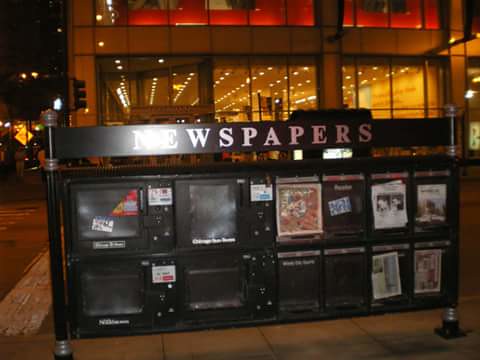The photo captures a nighttime urban scene featuring an unattended, coin-operated newspaper vending machine mounted on two sturdy metal poles. The newspaper stand, aligned horizontally, has a large black metal sign at the top inscribed with "NEWSPAPERS" in bold white letters. Below this sign are 12 compartments with transparent glass or plastic windows, revealing their contents. On the left side, there are four larger compartments, most of which are empty, while one contains newspapers. The right side holds eight smaller compartments, with only three or four filled with newspapers, leaving the others vacant. The background shows a multi-story building illuminated by both interior and exterior lights, with yellow lights dominating the inside and red hues noticeable at the upper-level windows. The sky in the top left corner is dark, emphasizing the nighttime setting. This street corner, likely in a metropolitan area, is characterized by its ambient city lights, contributing to the overall urban atmosphere.